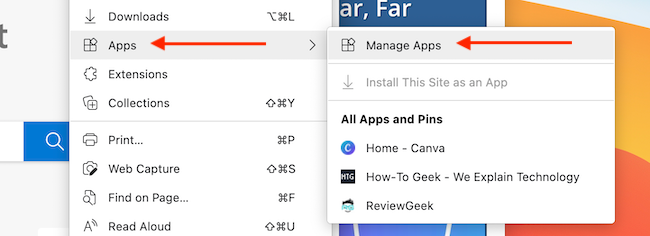In this image, we observe two prominent pop-up menus from a menu bar interface. 

On the left pop-up menu, the title "Downloads" is displayed at the top. The menu lists several options vertically: "Apps," "Extensions," "Collections," "Print," "Web Capture," "Find on Page," and "Read Aloud." Each of these options is accompanied by an icon to its left. Specifically, the icons are as follows: a downward arrow for "Downloads," four small squares for "Apps," a puzzle piece for "Extensions," a plus sign for "Collections," a printer for "Print," a camera for "Web Capture," a magnifying glass over a paper for "Find on Page," and an 'A' icon for "Read Aloud." A red arrow pointing to the word "Apps" indicates user focus or selection.

On the right pop-up menu, the title "Manage Apps" appears at the top, with another red arrow pointing towards it. Below the "Manage Apps" section, there are further options including "Install this site," "All apps and pins," "Home Cabinet," "How to Geek We Explain Technology," and "Review Geek."

In the background on the right side of the image, a gradient of warm colors transitioning from orange to dark orange is visible, adding visual context to the interface.